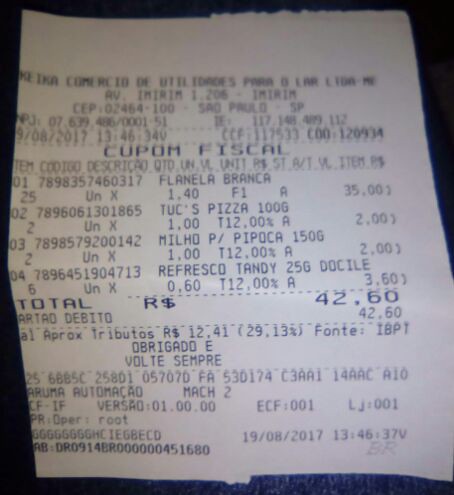This image depicts a white, rectangular receipt that is slightly bent towards the bottom middle, turning downwards to the right. The text on the receipt is printed in black. At the top of the receipt, although somewhat faded and difficult to read, it features the address and phone number, followed by the words "CUPOM FISCAL." The receipt likely originates from a foreign country, potentially Brazil, given the use of terms such as "Sao Paulo" and "Tributos." The listed items include Flanella Branca, Tux Pizza, Milo, Pipoca, and Refresco Tandy, with item prices totaling R$42.60. The receipt also notes tributes of R$12.41. A credit card was used for the transaction, which took place on August 19, 2017, at 1:46 PM. The overall receipt is not in perfect condition, showing signs of rough edges and slight folds.